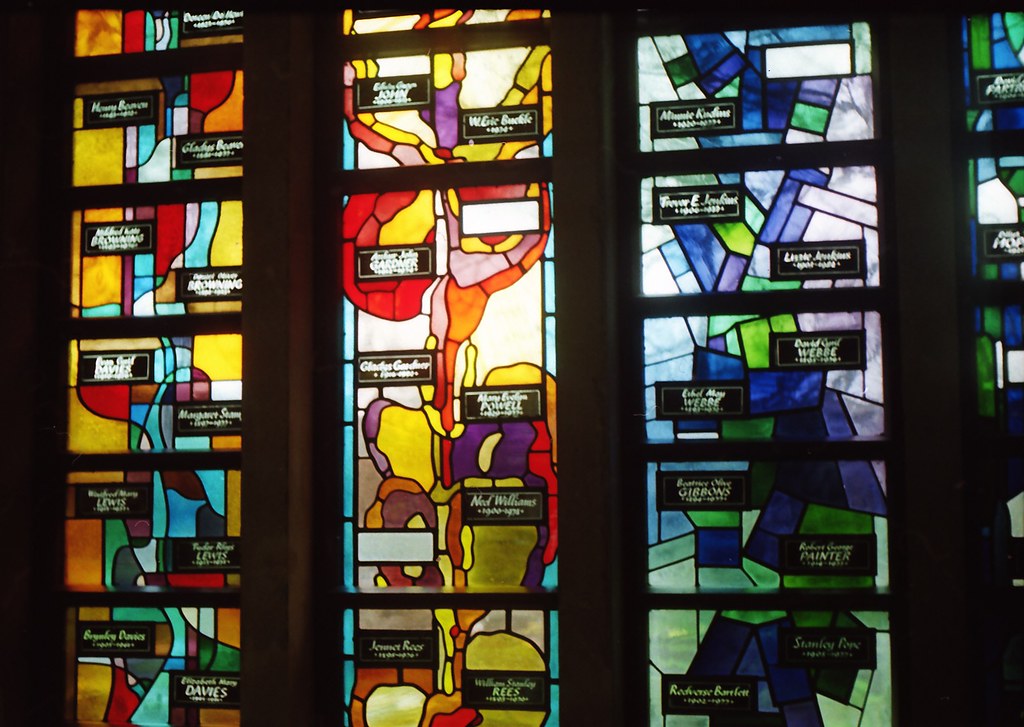This image depicts a beautiful wall comprised of stained-glass windows arranged into four distinct columns, though three columns are the most prominently visible. The stained glass is segmented into various geometric shapes, predominantly rectangles and squares. 

The leftmost column features a majority of yellow, orange, and blue hues, segmented into small rectangles. Each section features two smaller black rectangles inscribed with names and dates, possibly memorials or dedications. There's a mixture of red, blue, green, and white colors throughout this column's design.

The second column showcases a central giant rectangle with surrounding squares, presenting a vibrant palette of red, yellow, blue, and white. Unlike the first column, it has fewer segments dedicated to names or memoriams.

The third column mirrors the pattern of the first, including the names and small black rectangles, but focuses more on green, blue, pink, and white colors.

The fourth column, primarily dark blue with light blue, green, purple, and white accents, features intricate designs including butterflies — a red and pink butterfly and a purple and yellow one. This column, like the others, houses various names and memorials.

Overall, the stained glass wall is a colorful tribute with an intricate interplay of hues and memorial inscriptions scattered throughout the varying segments.